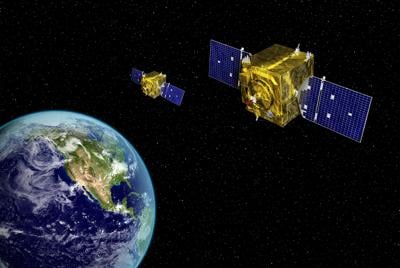This captivating image showcases a detailed satellite photograph capturing another satellite in the act of photographing Earth. The main satellite, positioned closer to the camera, is prominently in the foreground, while a second satellite can be seen in the background, both orbiting the planet. Earth is partially visible, occupying the lower-left corner of the frame with about one-third of its sphere cut off. The visible portion of Earth appears to depict the southern region of the United States, viewed from the perspective of the Pacific Ocean. Notably, the planet is slightly off-center within a rectangular section of the image, surrounded by the vast, stark blackness of space. Interestingly, the absence of any visible stars adds a certain intrigue to the composition, raising questions about the image's authenticity and the typical portrayal of the cosmos.